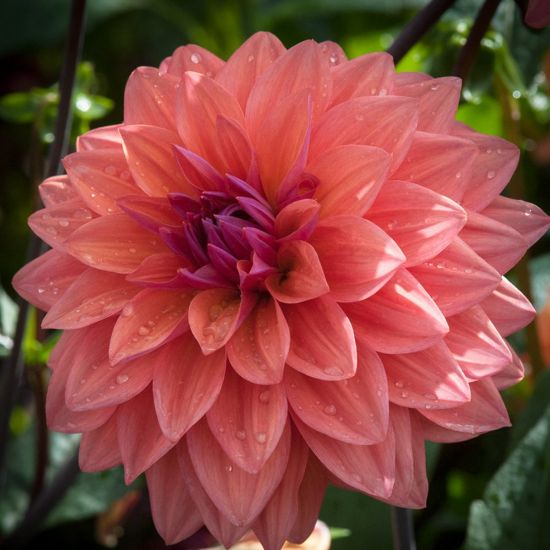This image is a highly detailed, close-up shot of a blooming flower prominently featuring a rich array of pink hues. The composition captures the intricate layers of petals that cascade from the outer edge towards the center, where they narrow dramatically. The outer petals exhibit shades of light to dark pink, transitioning into deeper purple tones as they gather tightly in the middle, suggesting the structure of a dahlia. Dew adorns the petals, adding a glistening effect that enhances the flower's vivid colors. The bloom is dense and sizable, about an inch thick and two inches around. Surrounding the flower, the backdrop includes slightly out-of-focus green foliage and large, oval-shaped leaves growing from a sturdy green stem, which provides a natural contrast and emphasizes the flower's vibrant centerpiece.